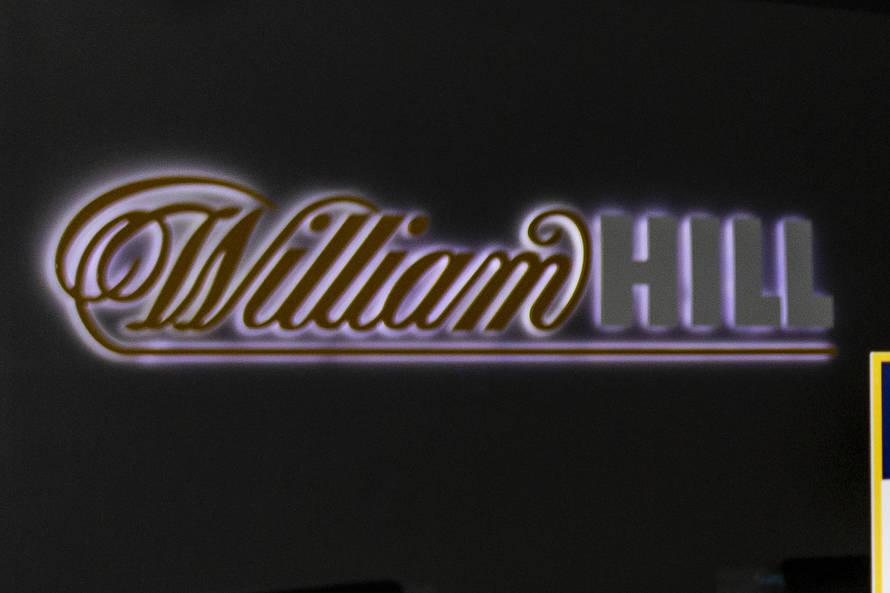The image features a digitally created logo on a black background, prominently displaying the name "William Hill" at its center. The word "William," written in an elegant, cursive script reminiscent of old English calligraphy, appears in a deep burgundy or brown color with white highlights and intricate swirls at the beginning of the 'W' and end of the 'M'. Below, the word "Hill" is printed in bold, 3D-style block letters, rendered in gray with white borders. The cursive script from "William" extends below, creating an underlining swirl that connects the two names. In the right corner of the image, there is a small, unidentifiable yellow streak descending diagonally, adding a minor visual element to the overall design. This logo seems to be an advertisement or brand decal for "William Hill."